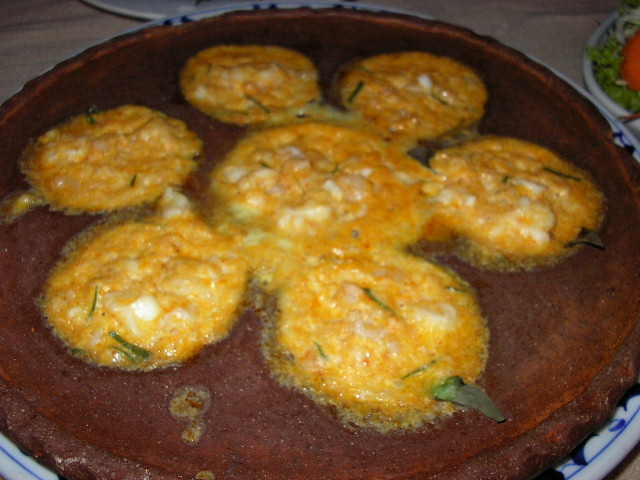On a rustic brown wooden slab, which is set atop a larger white plate with blue markings, there are seven round, battered or breaded objects. These golden-brown items have green specks, resembling herbs or parsley, and appear to contain melted, possibly cheesy ingredients with white curds. They look chunky and fried or grilled, giving them a browned, crispy exterior. The setting includes another smaller plate visible to the right, holding something red and green, and everything rests on a gray dinner table.